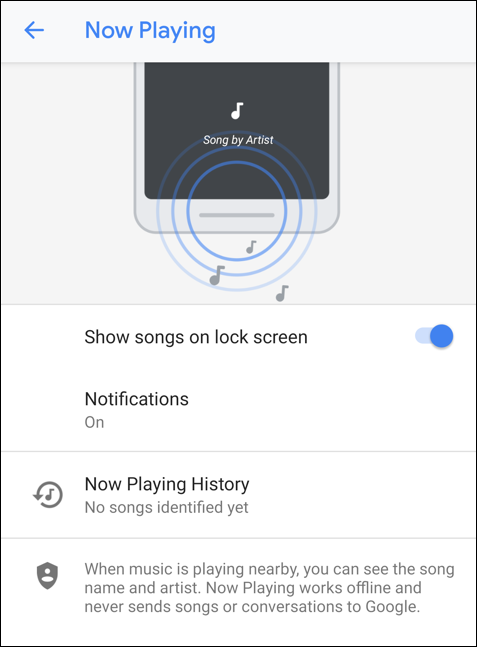The image is a rectangular graphic divided horizontally into two sections: the top half is gray, and the bottom half is white.

**Top Half:**
- **Upper Left Corner:** Features a blue arrow pointing left with the text "Now Playing" in blue.
- **Center:** Displays a photo of the top half of a cell phone, with a white music note icon and the text "Song by artist" in gray on the phone's screen.
- **Below Phone Image:** Contains three concentric circles overlapping the bottom of the cell phone image and extending into the gray area, adorned with black music notes positioned between the lines.

**Bottom Half:**
- **Main Text:** "Show songs on lock screen" in black at the top.
- **Toggle Button:** Situated beneath the text, the button has a gradient from light blue on the left to a dark blue circle on the right, indicating it is turned on.
- **Notifications Section:**
  - The word "Notifications" appears in black with "On" in gray below it.
- **Now Playing History Section:**
  - An icon accompanies the text "Now Playing history" followed by "No songs identified yet" in gray.
- **Additional Information:**
  - An icon resembling a shield with an emblem of a person inside is displayed next to the text, "When music is playing nearby, you can see the song name and artist. Now Playing works offline and never sends songs or conversations to Google."